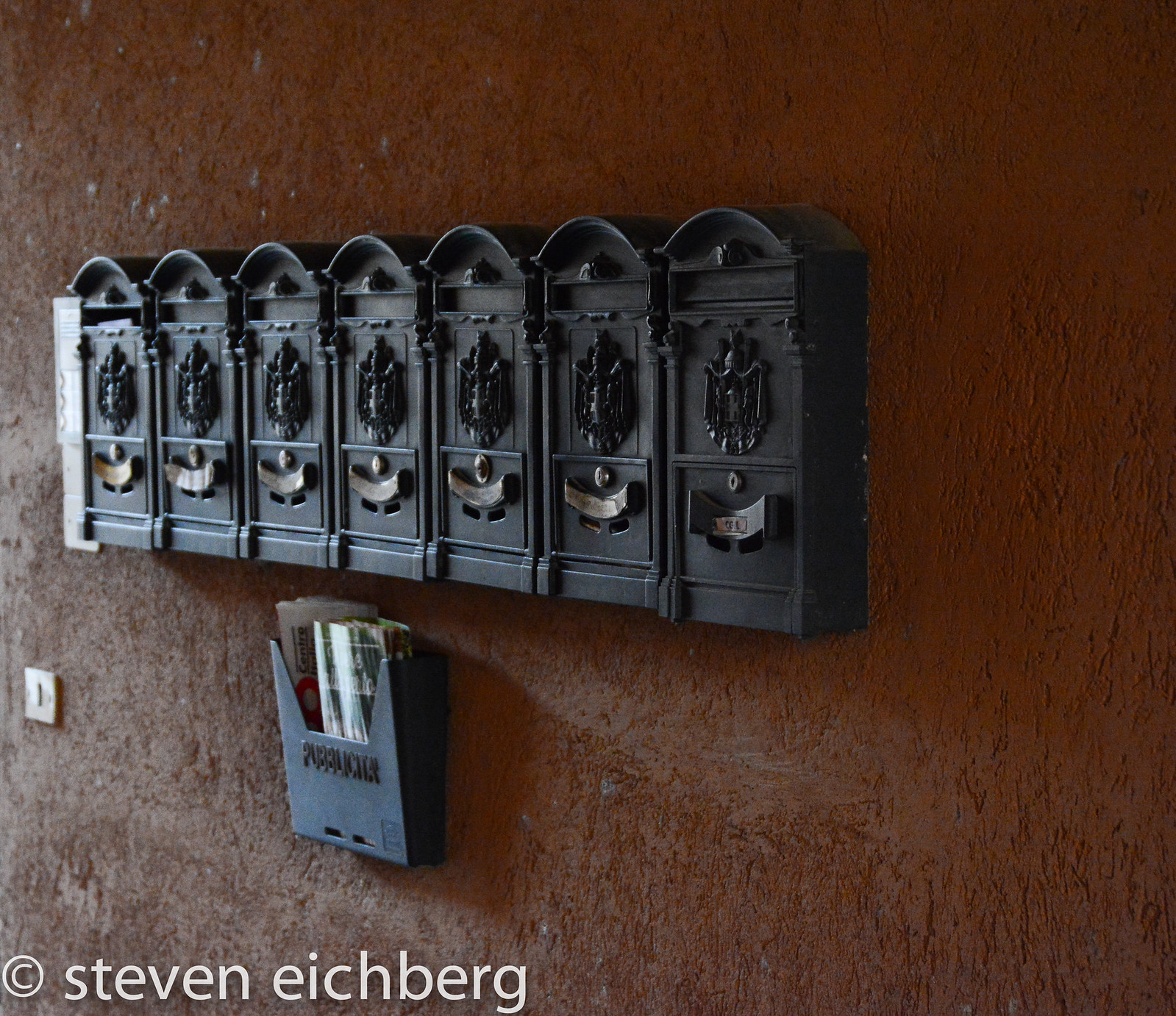The photograph showcases seven old-fashioned, Victorian-era letterboxes mounted horizontally on a textured, dark reddish-brown stucco wall. Each mailbox is made of dark gray or black metal with a glossy coat of arms logo on the front and a silver arch at the bottom, featuring small silver knobs and mail slots at the top. Below the row of letterboxes, a black container with the word "Publicator" in black lettering holds newspapers and documents, including a paper labeled "Contra." On the wall's bottom left corner, "C. Stephen H. Becker" is inscribed in white, and a white wall switch is visible in the left corner of the image. The left side of the photograph is more illuminated, giving a slight angle perspective that makes the mailboxes appear progressively smaller.